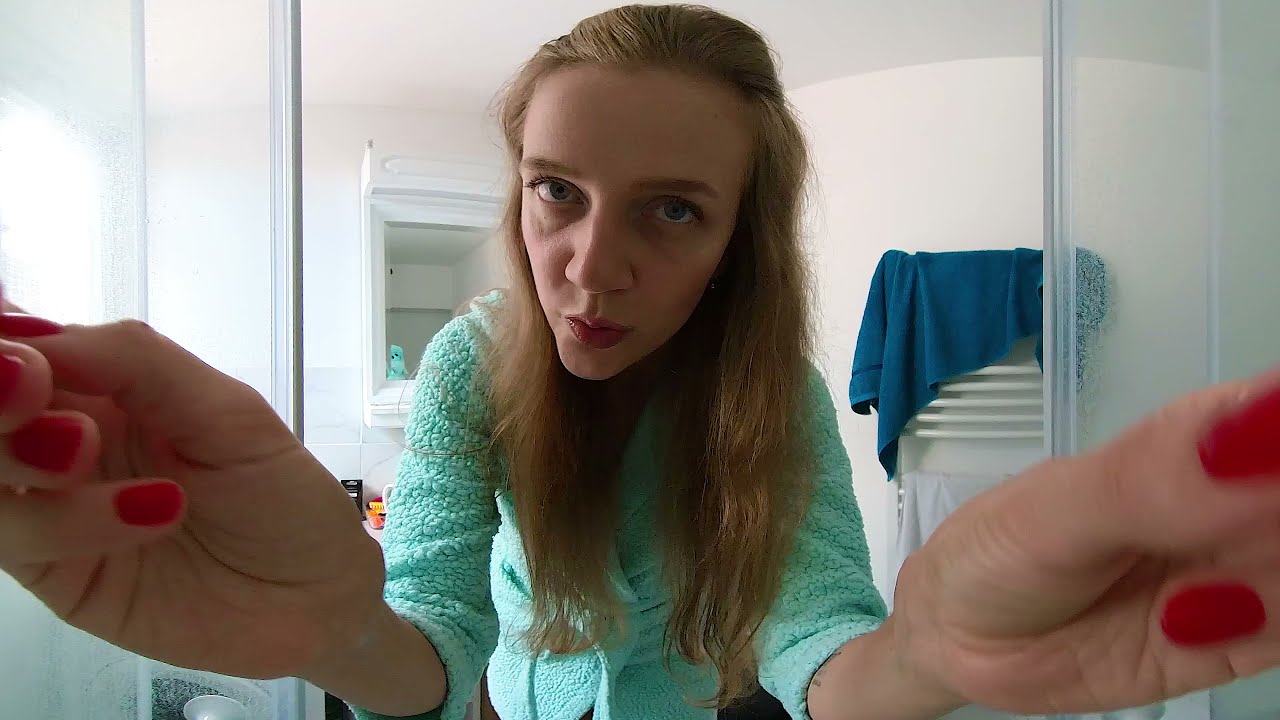A woman in her mid-30s with blue eyes and blonde hair, parted slightly to the left and cascading down to her stomach, is the focal point of the image. She appears to be taking a selfie, staring directly at the camera with her lips puckered as if blowing a kiss. She is wearing a light green sweater or robe that closes in the front and extends just below her elbows. Her hands, adorned with bright red fingernails, reach towards the camera, appearing much closer than her face. She stands in what seems to be a bathroom setting. Behind her, on her right side, a blue towel hangs on a rack against a white wall. The scene also features opaque shower doors with silver frames on both sides of the woman. To her left, there’s a square hole in the wall with a white frame and back. The image is set indoors, possibly in the middle of the day, as suggested by the vibrant lighting and subtle colors such as tan, light blue, off-white, yellow, black, and pink that complement the overall tableau.